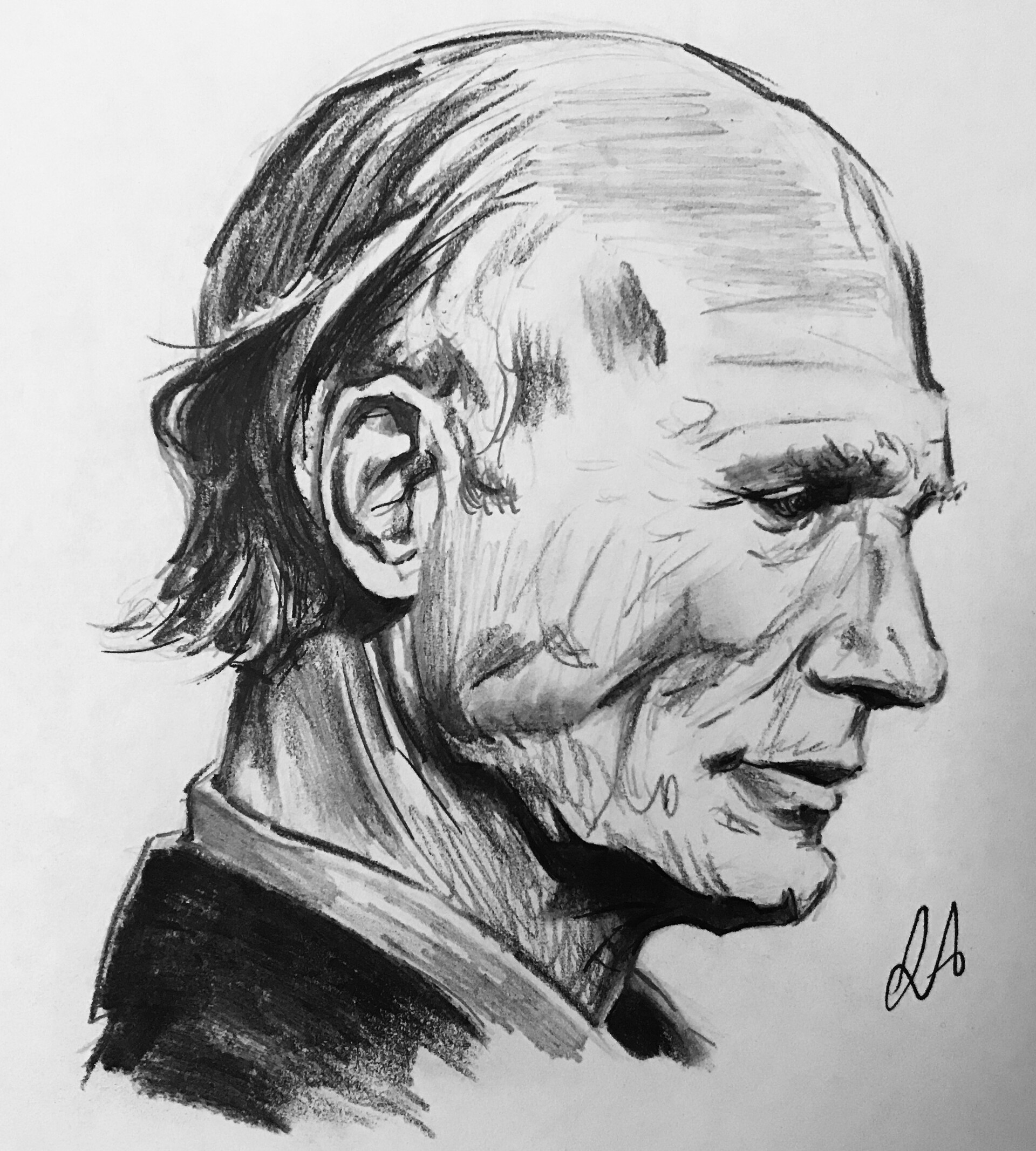This black and white sketch appears to be a detailed charcoal portrait of the renowned actor Ed Harris. The image captures Harris in a side profile, facing to the right with his gaze directed slightly downward. The meticulous artwork highlights his balding head with sparse, wavy hair towards the back, some of it tucked behind his ear. His facial features are sharp and craggy, with a pronounced bony nose, sunken cheeks, deep wrinkles, and a pointy chin. Thick, thin eyebrows convey a concerned expression. His mouth is slightly open, giving him a somewhat somber look. Harris is depicted wearing a jacket over a light-colored collared shirt. The background is a light gray, enhancing the contrast and intricate shading, with dark areas interspersed with subtle white highlights. In the bottom right corner, an artist's signature with what appears to be initials "DA" is visible.